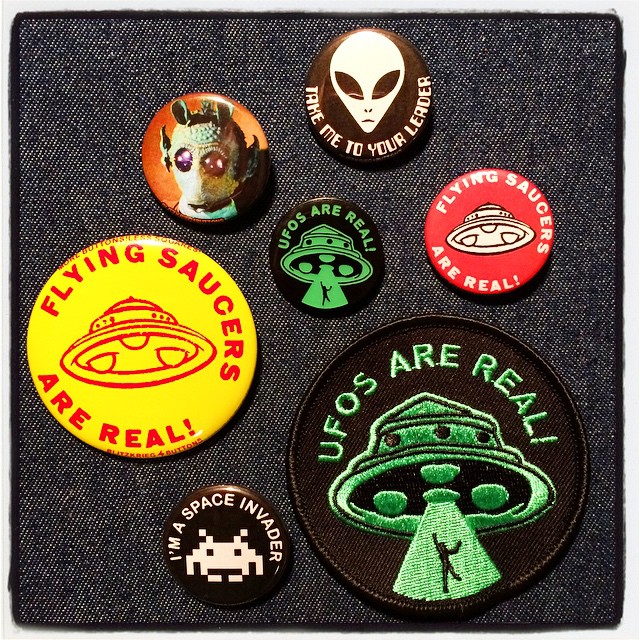This image shows a collection of seven round pins and patches of various sizes, neatly arranged on a square piece of dark blue denim fabric with white speckles. At the top is a brown pin featuring a white alien face with the text "Take me to your leader." Directly below this, on the left side, is a pin with an image of Greedo from Star Wars. Centrally located is a pin with green text on a black background that reads "UFOs are real," accompanied by an image of a flying saucer shining a beam of light on a man. To the right of this pin is a red pin with the text "Flying saucers are real" and a flying saucer in the center. Below this, in the bottom left, is a yellow pin with the same red text "Flying saucers are real" and a red flying saucer. Adjacent to it is a small black pin that says "I'm a space invader," featuring a character from the 80s video game Space Invaders. Finally, at the bottom is the largest item: a round black patch with the text "UFOs are real" and the same flying saucer image, featuring a beam of light on a human silhouette. The pins and patches exhibit a slight reflection from the lighting, adding a cohesive, captivating display.